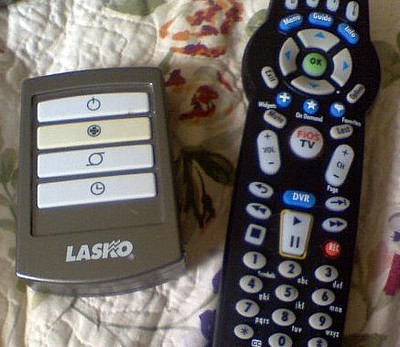This close-up photograph features two distinctive remote controls lying on a slightly quilted, off-white blanket adorned with floral patterns, particularly red and green hues that resemble cherries with leaves. The left remote is small, rectangular, and dark gray, designed for a fan by the brand 'Lasco,' as indicated at its bottom. It has four buttons: the top one is white with a circular symbol, followed by a beige button with a blue plus sign, a white button featuring a circle with lines on the top and bottom, and a bottom button with a clock icon. The right remote is a regular black TV remote labeled "FIOS TV" on its central button, with a blue "DVR" button underneath. It is equipped with various white and blue buttons for navigating menus, numbers, and other TV functionalities.